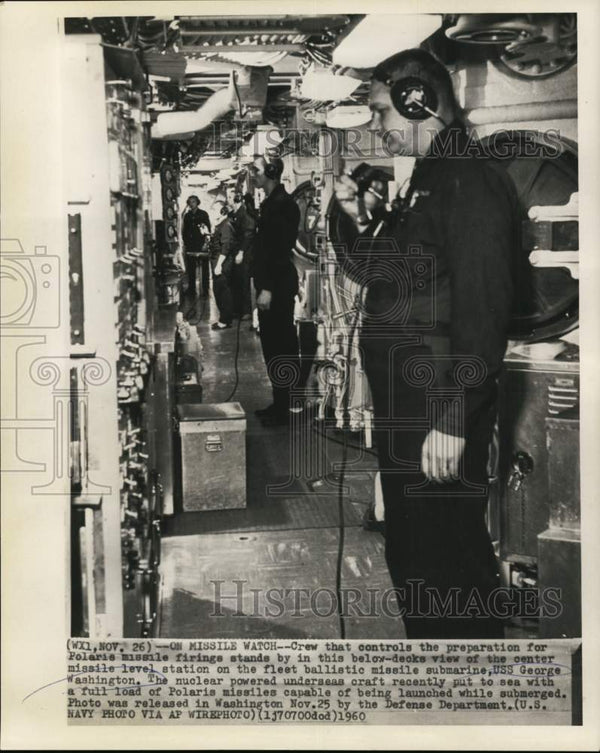This vintage black-and-white photograph, likely from the 1950s or 1960s, captures a moment below deck on the Fleet Ballistic Missile Submarine USS George Washington. The image shows a group of sailors standing in a row, about ten feet apart, each dressed in black jumpsuits and wearing headsets with microphones held up to their mouths. These men are positioned in front of panels densely packed with various buttons and switches, attentively monitoring and ready to control the preparation for Polaris missile firings. This below-deck view, identified as the center missile level station, is illuminated by large fluorescent lights overhead, contributing to the stark, utilitarian environment typical of a military submarine. The caption beneath the image indicates that this scene was part of the submarine's operations as the vessel embarked on a mission carrying a full load of Polaris missiles, which are capable of being launched while submerged. The photograph was released in Washington by the Defense Department on November 25, 1960, and is credited to the U.S. Navy via AP wire.